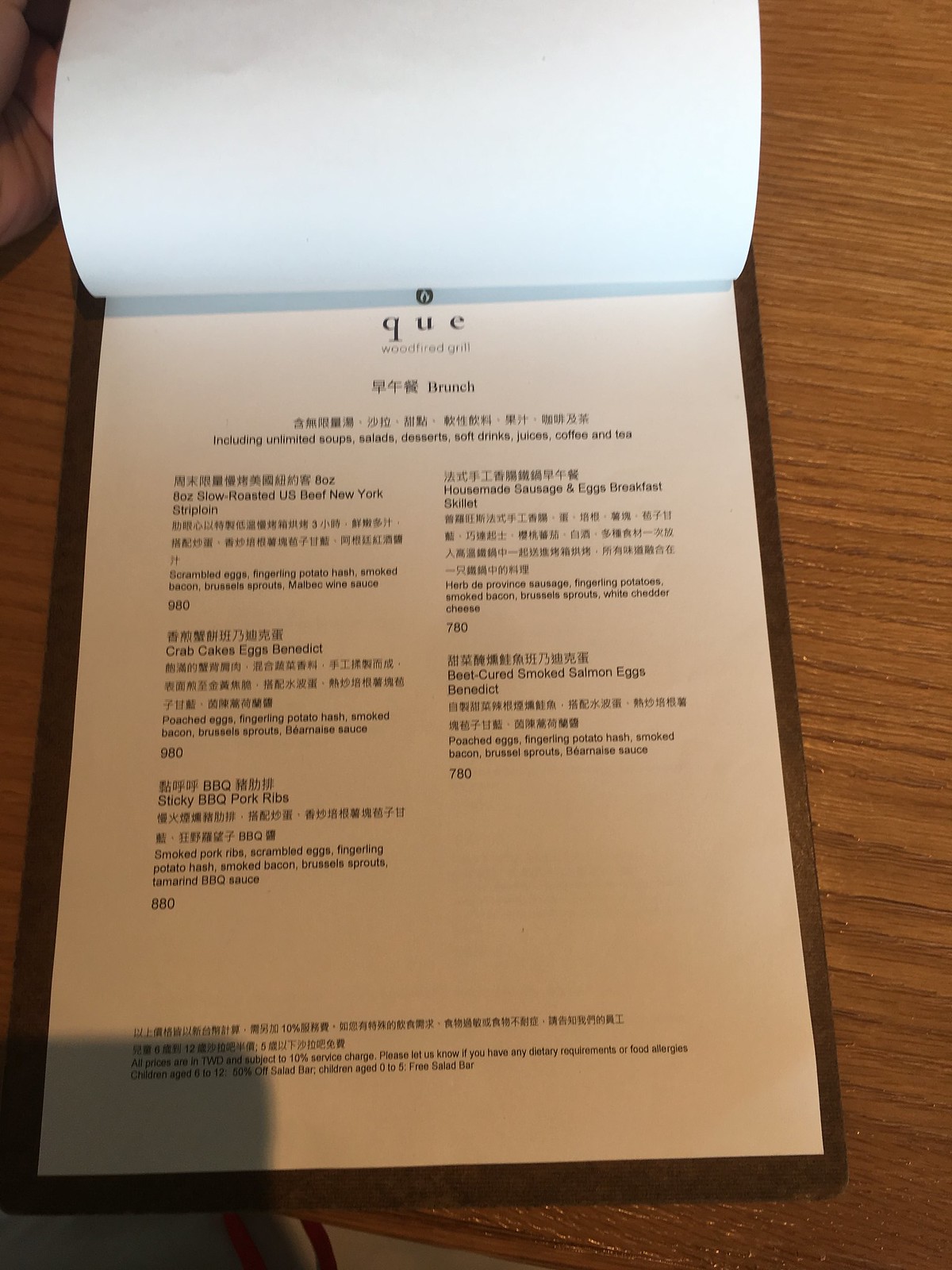In this photograph, we see a meticulously crafted menu from Q-UE Woodfired Grill, set against a light brown, textured wooden table. The menu is affixed to a polished, darker brown clipboard, enhancing its rustic elegance. A white sheet of paper bears the detailed menu, with a hand visible in the frame, lifting a page of the menu for a clearer view of the selections.

The heading boldly proclaims "Q-UE Woodfired Grill" with the subheading "Brunch" and highlights the inclusive offerings of unlimited soup, salads, desserts, soft drinks, juices, coffee, and tea.

### Featured Dishes:

- **8 oz. Slow-Roasted US Beef New York Strip Loin**:
  - Accompaniments: Scrambled eggs, fingerling potato hash, smoked bacon, Brussels sprouts, and Melibic wine sauce
  - Price: 9.80 TWD

- **Crab Cakes Eggs Benedict**:
  - Accompaniments: Poached eggs, fingerling potato hash, smoked bacon, Brussels sprouts, and Béarnaise sauce
  - Price: 9.80 TWD

- **BBQ Sticky Pork Ribs**:
  - Accompaniments: Smoked pork ribs, scrambled eggs, fingerling potato hash, smoked bacon, Brussels sprouts, and Tamarind BBQ sauce
  - Price: 8.80 TWD

- **House-Made Sausage and Eggs Breakfast Skillet**:
  - Components: Herb de Provence sausage, fingerling potatoes, smoked bacon, Brussels sprouts, and white cheddar cheese
  - Price: 7.80 TWD

- **Beet-Cured Smoked Salmon Eggs Benedict**:
  - Accompaniments: Poached eggs, fingerling potato hash, smoked bacon, Brussels sprouts, and Béarnaise sauce
  - Price: 7.80 TWD

At the bottom of the menu, it is noted that all prices are listed in TWD and subject to a 10% service charge. There is also a considerate notice for dietary restrictions or food allergies. Special offers include a 50% discount on the salad bar for children aged 6-12, and a free salad bar for children aged 0-5.

Additionally, the entire menu is translated into Japanese, ensuring accessibility for a diverse clientele. The thoughtful design and detailed descriptions evoke an air of sophistication and attention to detail, reflecting the restaurant's commitment to providing an exceptional dining experience.